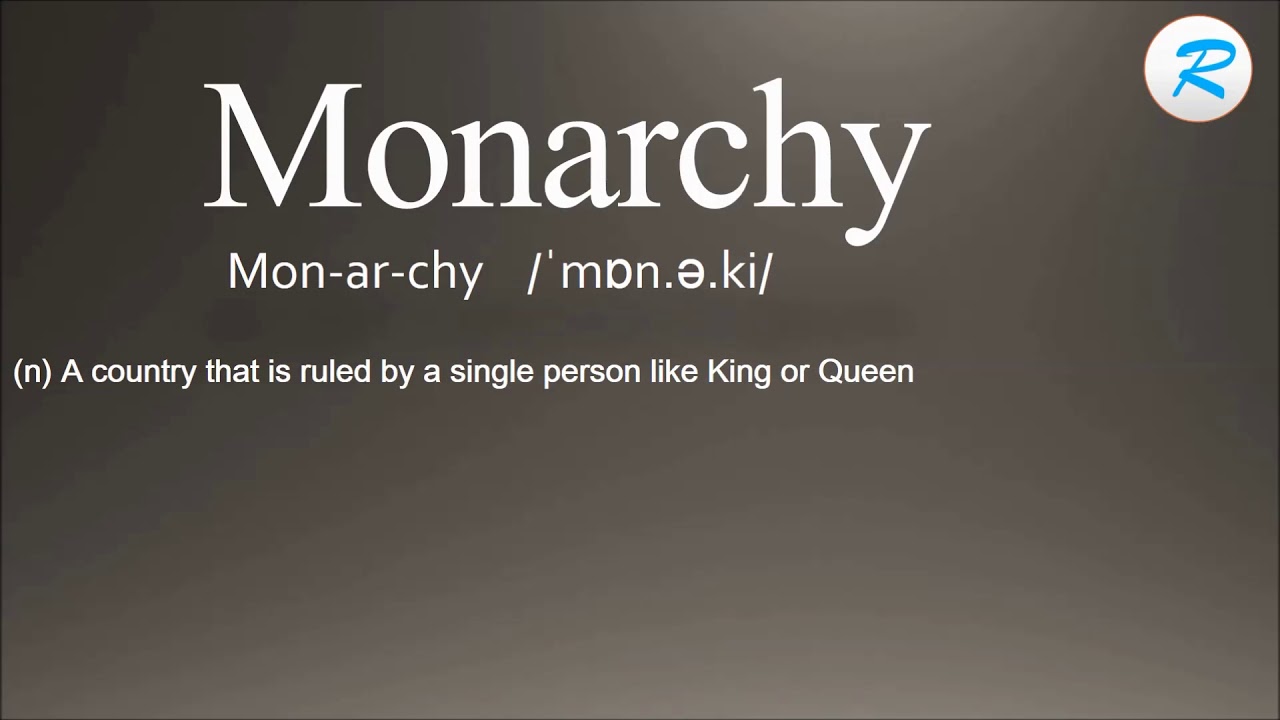The image appears to be an educational slide with a gradient gray background, darker on the edges and lighter towards the center, simulating a light source from the upper right. Dominating the upper portion of the image is the word "Monarchy" in large, bold, white font, with the first letter capitalized. Directly beneath it, the word is phonetically broken down into syllables, first as "mon-ar-key" and then as "/mɒn.ə.ki/," both in white text. Further down, contained in parentheses, there's an "N" indicating the part of speech (noun), followed by the definition in white text: "a country that is ruled by a single person like a king or queen." In the upper right corner of the image, there is a white circle with a blue, cursive uppercase 'R' centered inside it. This could represent a logo or a dictionary reference marker.